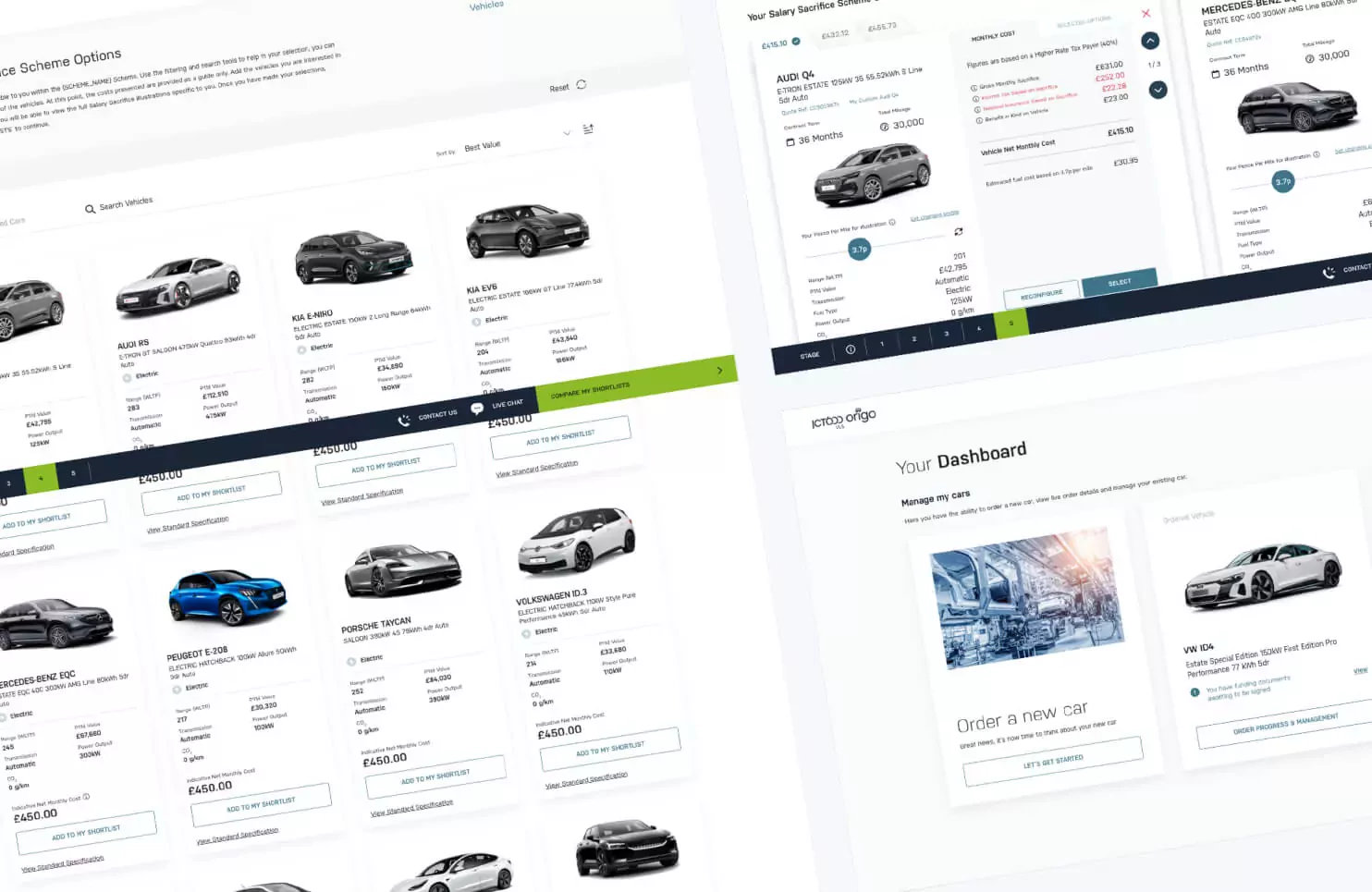The image appears to be a spread from a car brochure, viewed at an angle and tilted slightly to the left, resulting in all four corners being cut off. The background is white. On the top left side, bold black lettering reads "Scheme Options," beneath which is smaller, regular text. The page prominently features multiple rows of cars.

There are four cars in the top row and another row of four cars in the middle, separated by a horizontal navy blue line with green embellishments. The third row at the very bottom only reveals a small portion of one car and two complete automobiles.

On the right side of the spread, the visible section showcases three distinct areas displaying cars. Another horizontal blue line divides this section from the footer, which reads "Your Dashboard." Below this, text likely states "Manage My Cars," accompanied by two car images. This brochure includes multiple brands, with discernible logos indicating Porsche, Volkswagen, and Audi, each accompanied by detailed information about the vehicles.